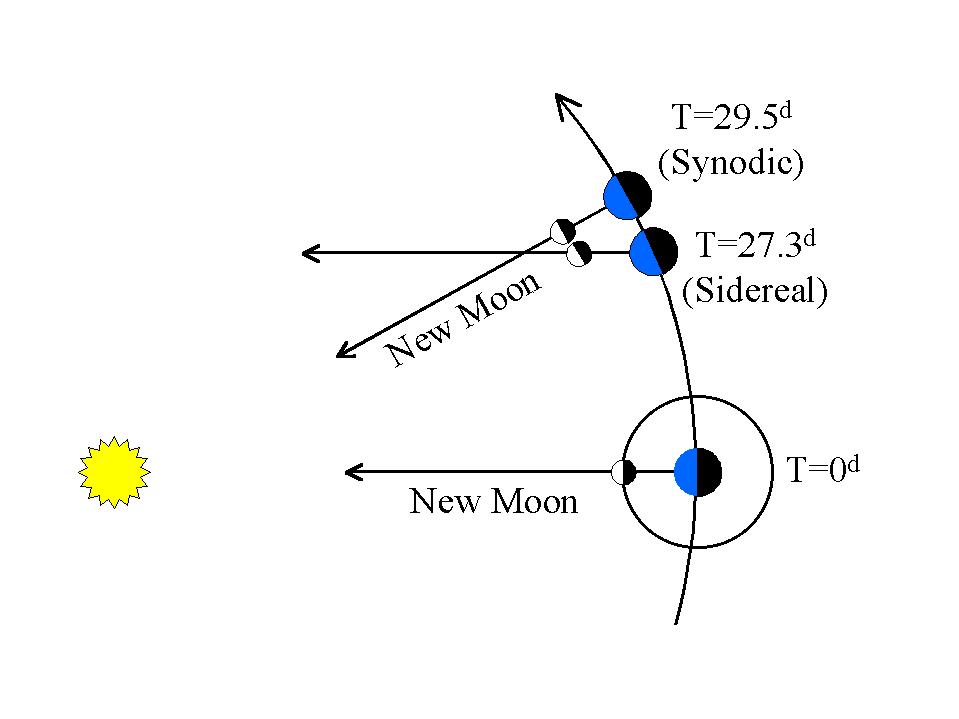A detailed scientific chart on a white background illustrates the relationship between the Moon and the Sun. The chart utilizes a black, blue, and yellow color scheme typical of computer-generated graphics. Prominently on the left-hand side, a yellow circle with a zigzag edge, reminiscent of a metallic seal on a diploma, represents the Sun. An arcing black line, which curves from the bottom to the top with an arrow pointing to the top left, depicts the Moon's orbital path. 

Along this arcing line, three half-blue, half-black circles represent the Moon, with the blue side facing the Sun. This arrangement illustrates various lunar phases as viewed from Earth. Each circle has a black line emanating from it: the bottom one labeled "New Moon" points downwards, the middle one, unlabeled, points horizontally to the left, and the top one, also labeled "New Moon," points downwards. 

To the right of the chart, there is a notation “t = 29.5 d synodic,” indicating the average synodic month, or the time taken for the Moon to return to the same phase (approximately 29.5 days). The illustration includes multiple directional arrows and mathematical annotations, providing a detailed depiction of the Moon's positioning relative to Earth and the Sun, aimed at explaining the phases of the Moon and the process of new Moons through its orbital cycle.